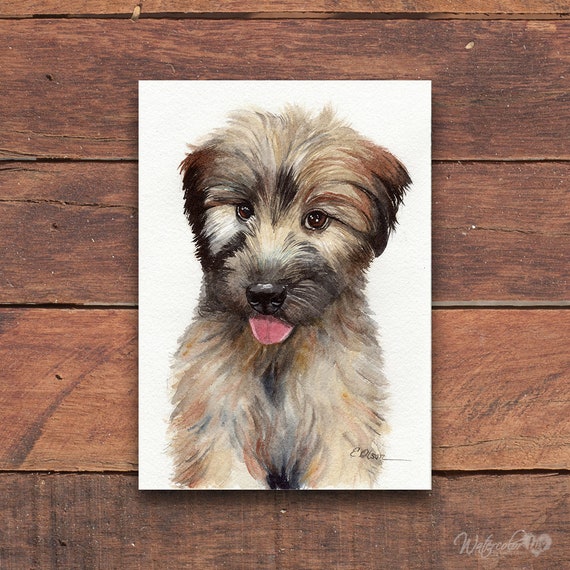This image captures an illustration of a fluffy dog rendered in an artistic watercolor style, placed on a white piece of paper. The paper rests on a medium to dark brown wooden table composed of four horizontal slats. The dog has a cute and expressive face, characterized by big brown eyes and a black nose, with its tongue playfully sticking out. Its fur is a mix of colors, including light and dark brown, gray, black, beige, and white, with noticeable brushstrokes and pencil marks adding texture and depth. You can see the dog from its shoulders to the top of its head, with small ears that hang down the sides of its face. The artist's signature is located in the bottom right corner of the illustration, and the photograph also features a semi-transparent watermark reading "watercolor" in script towards the corner of the image.